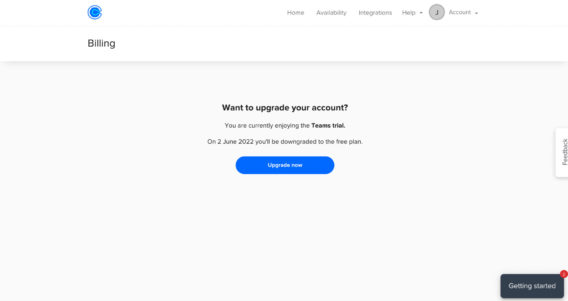Screenshot of a user interface from an unidentified web page with a focus on billing information and account management options. At the top left, the title "Billing" is prominently displayed. To the top right, navigation links labeled "Home," "Availability," "Integrations," and "Help" are clearly visible, followed by a gray circle icon resembling clock hands, indicated as the "Account" section.

A message informs the user about being currently on a Teams trial, which will revert to a free plan in June 2022 unless an upgrade is made. A noticeable dark blue, oblong button labeled "Upgrade Now" in white font is positioned beneath this message, prompting the user to upgrade their account.

In the bottom right corner, the words "Getting Started" are featured in white within a black box, with a small red circle at its top right edge. Additionally, a vertical white feedback tab is situated along the right edge of the screen.

This image solely consists of web page elements and contains no people, animals, plants, vehicles, or any other extraneous objects.